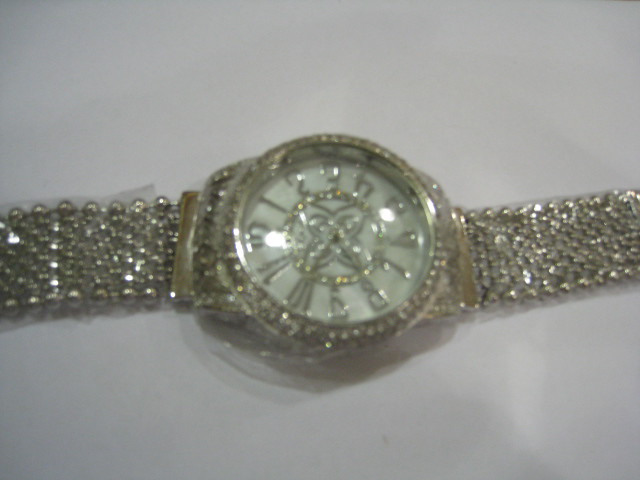In the slightly rectangular, horizontally oriented image, the background fades from white to off-white, providing a neutral canvas for the central object: a highly ornate wristwatch. The watch face is prominently featured in the center of the frame, with portions of the band visible extending horizontally on either side. The entire watch appears to be wrapped in a clear protective covering. The watch face itself is pristine white, adorned with goldish-silver numerals that elegantly mark the hours. The band is exquisitely textured, designed in a series of rows that resemble small, glistening beads, creating a visually captivating, sparkling effect that catches the light from various angles.